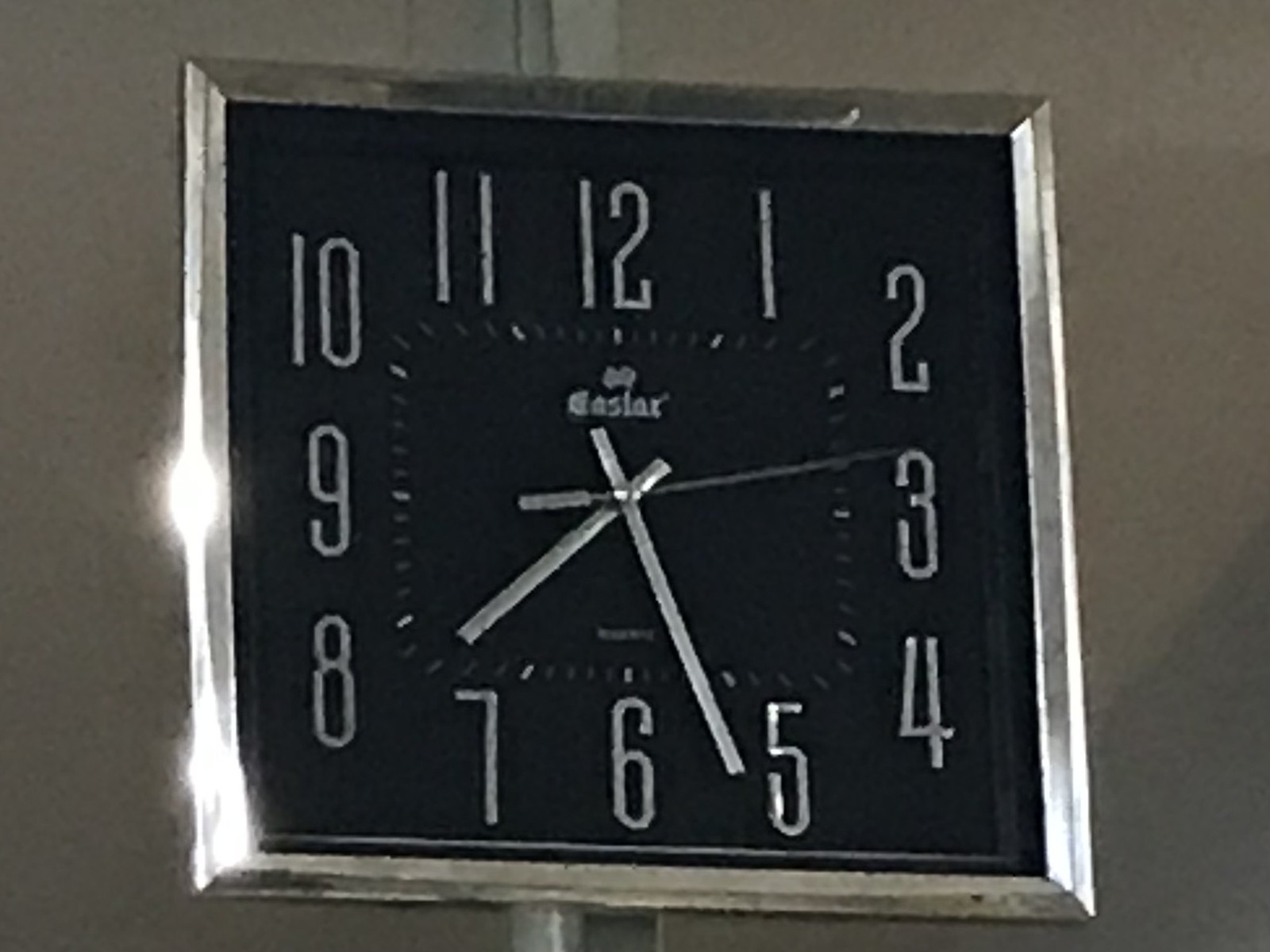This photograph features a square-shaped clock mounted against a grey backdrop. The image quality is slightly grainy, suggesting it is of lower resolution. The clock is adorned with a chrome bevelled border that adds a touch of modern sophistication. The clock face is black, contrasting sharply with the white Arabic numerals positioned around its perimeter. 

The clock hands are made of metal, with the minute hand being long and thin, while the shorter hour hand shares a similar rectangular shape. Additionally, a slender metal second hand is captured pointing approximately halfway between the 2 and the 3. The numerals on the clock face are rendered in a silvery chrome hue, harmonizing with the clock’s overall metallic theme. Minute markers are also present, subtly arranged inside the numerical ring, enhancing the clock’s precision and functionality.